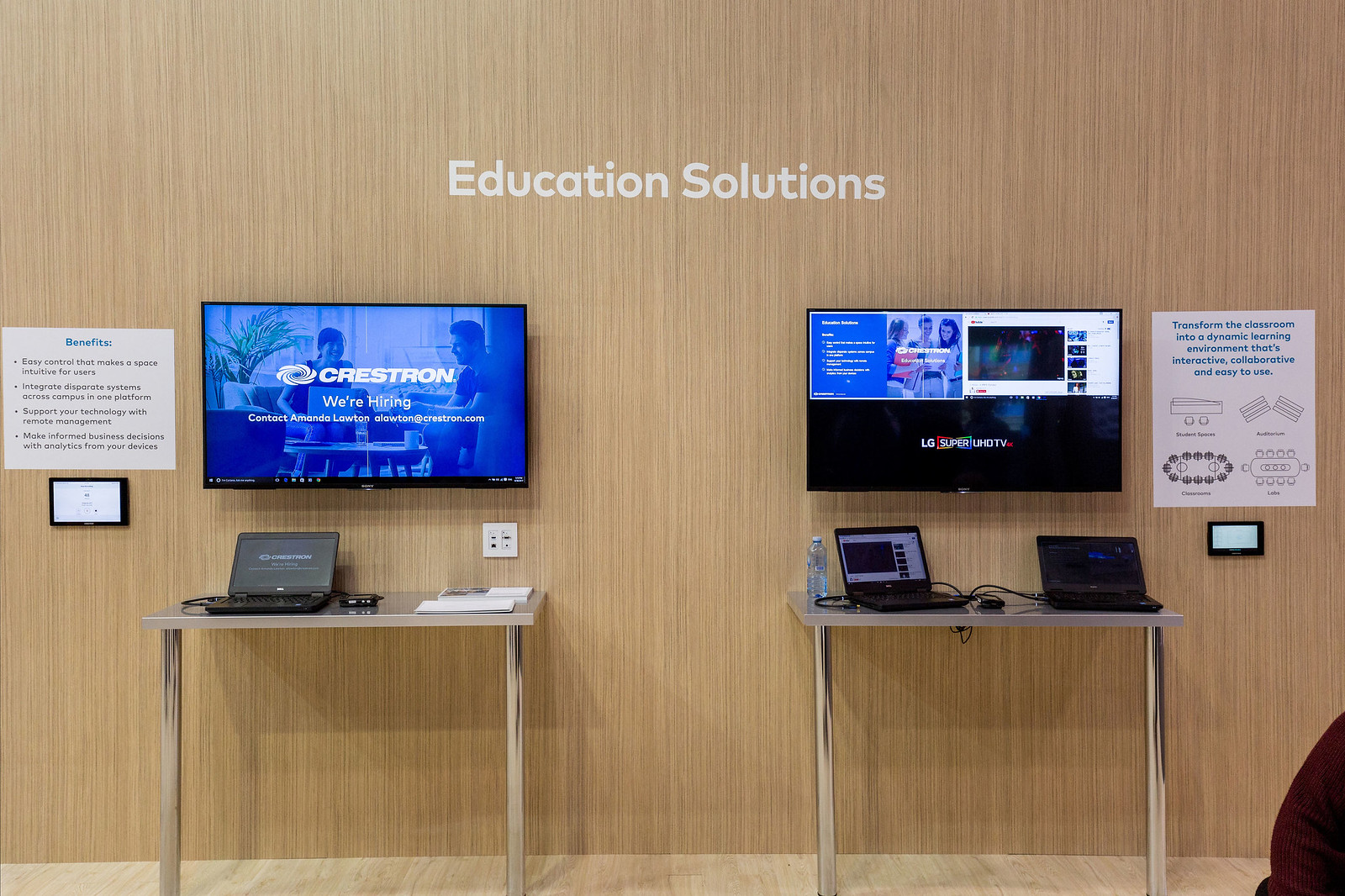The image depicts a light-colored wooden paneled wall with a hardwood floor. Positioned approximately three-quarters up the wall are two wall-mounted screens or small televisions, one on the left and one on the right. Above these screens, in white text, is the phrase "Education Solutions." Below the screens, there are two silver metal desks, each supported by two legs. 

The right desk holds two laptops, while the left desk has one laptop. On the left screen, in white text, the word "Crestron" appears, followed by "We're hiring. Contact Amanda Lawton, alawnton@crestron.com." Additionally, there are some indecipherable writings and small pictures hanging on both sides of the wall, contributing to the overall setup.